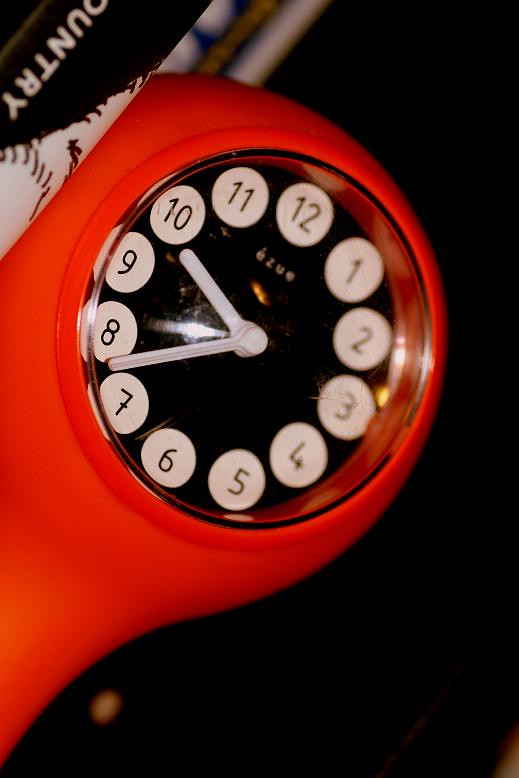The photograph, likely taken with a phone due to its vertical orientation, features a predominantly black background, possibly a wall, that is difficult to discern. Centered in the image, there is an orange clock made primarily of orange plastic. The clock has an elongated oval shape, wider than it is tall, with a curved and glossy glass covering its face. 

The clock itself is branded "Iswear," and its face has a black background with white circular markings detailing the hours, numbered from 1 through 12 in black. The clock's hands are white plastic, with the minute hand positioned between the 7 and 8 and the hour hand pointing almost towards 10, indicating a time close to 9:35. 

In the top left corner of the image, there is a partially visible object that could be a pole, a glove, or the handle of a bat, featuring the word "country" on it. The overall composition suggests that the photo was taken in a low-light environment, potentially a dimly lit room or a darkened area.